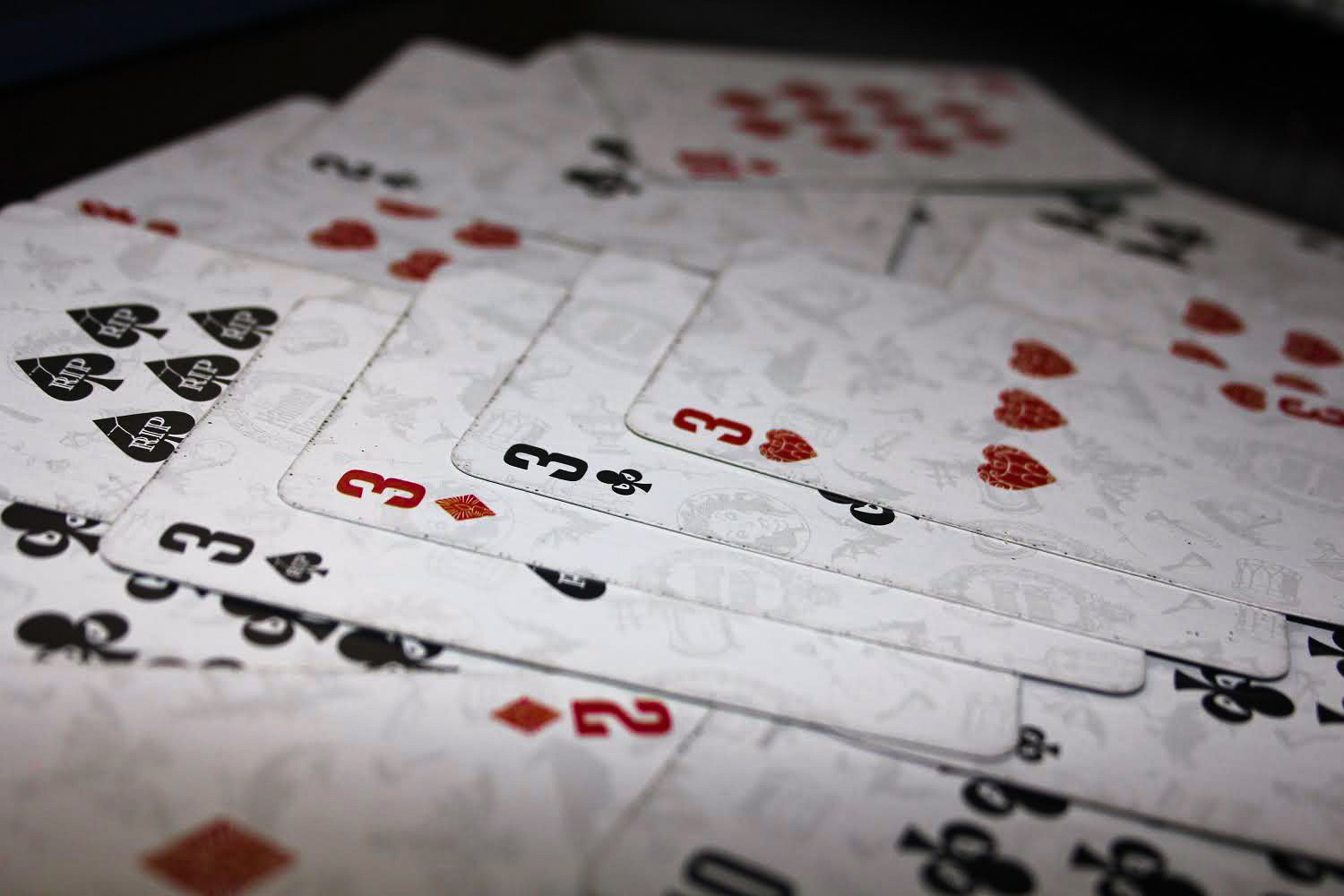The image captures a chaotic pile of playing cards, with the top few cards sharply in focus while the rest fade into a blur. The detailed designs on the cards extend beyond the standard suit icons of hearts, clubs, spades, and diamonds, featuring an eclectic mix of illustrations including an alien Medusa, a medical staff, a seal, a snare drum, and a boat, among others. The three prominently displayed cards are all threes, one from each suit, suggesting they belong to the same deck. Additionally, visible near the top are a two of diamonds, a two of spades, and a unique card bearing the spades symbol and the letters "RIP." The majority of the pile remains indistinct and unidentifiable, adding to the randomness and mystery of the assortment.